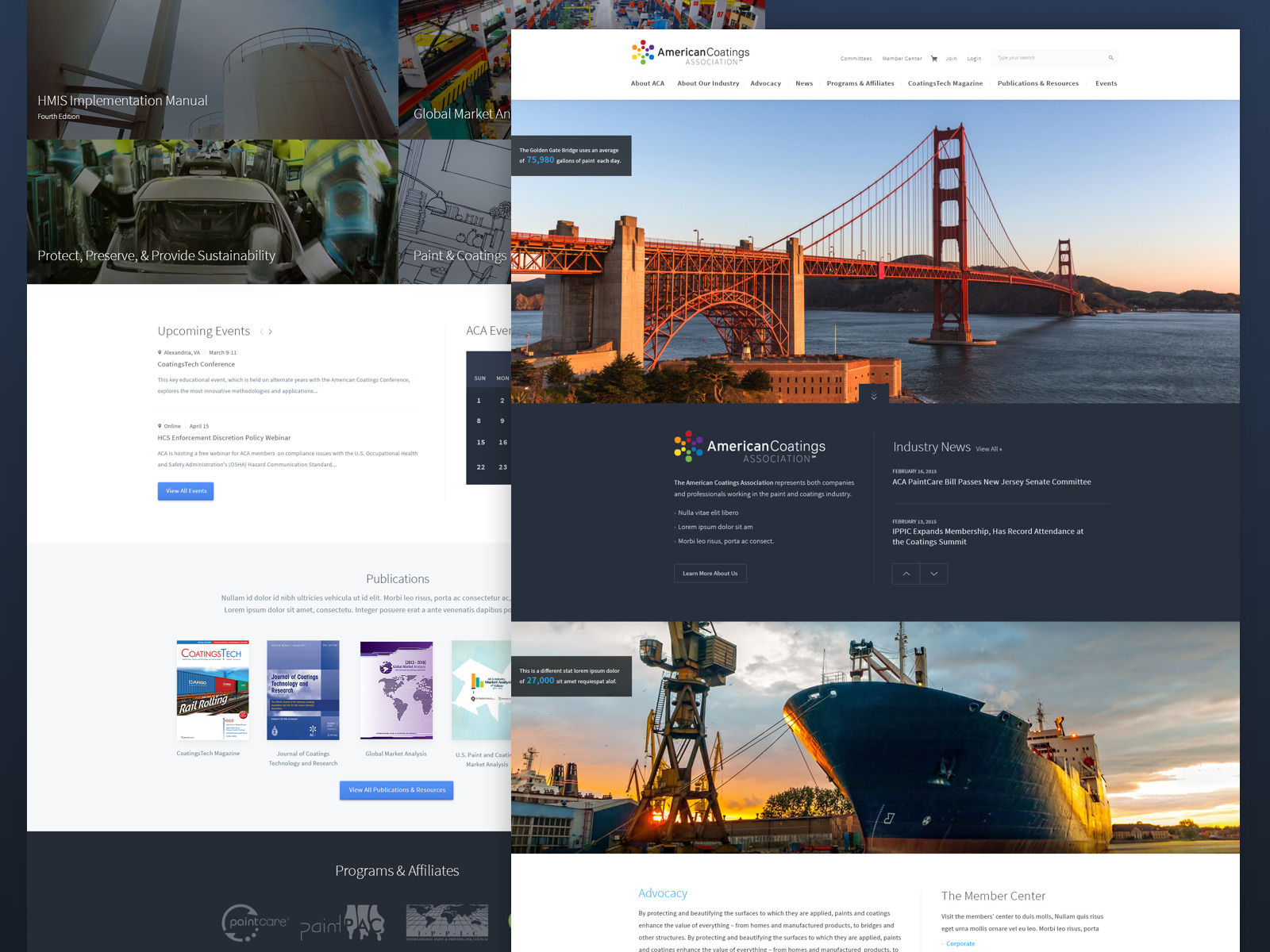This image is a composite screenshot of a webpage, meticulously edited to display both the top and bottom sections of the site simultaneously. In the background, the bottom half of the webpage is spread out, while a smaller overlay to the top right corner showcases the top section of the website.

The top portion features the website's masthead with the title "American Castings." Directly beneath the title is a navigation bar with various categories. Below this navigation bar, there is a large, striking photo of the Golden Gate Bridge, which dominates the visual space.

In the content area under the Golden Gate Bridge photo, the text reads "American Codings Association," followed by a brief description. To the right of this description is a section labeled "Industry News," accompanied by a couple of pertinent links. Further down this section are two arrow buttons, facing up and down, designed for scrolling through the content.

Below the "Industry News" and its scrolling section is an image of the imposing front of a commercial ship, adding to the maritime theme. Underneath this, there are two distinct sections. The left section appears to be an "About" section, while the right is designated as the "Member Center."

The background layer reveals the bottom of the webpage, featuring thumbnails of diverse items and a highlighted section titled "Upcoming Events." Additionally, on the bottom left, there are thumbnails of publications. The top overlay effectively covers the entire right side of the background, presenting a seamless blend of the top and bottom parts of the webpage.